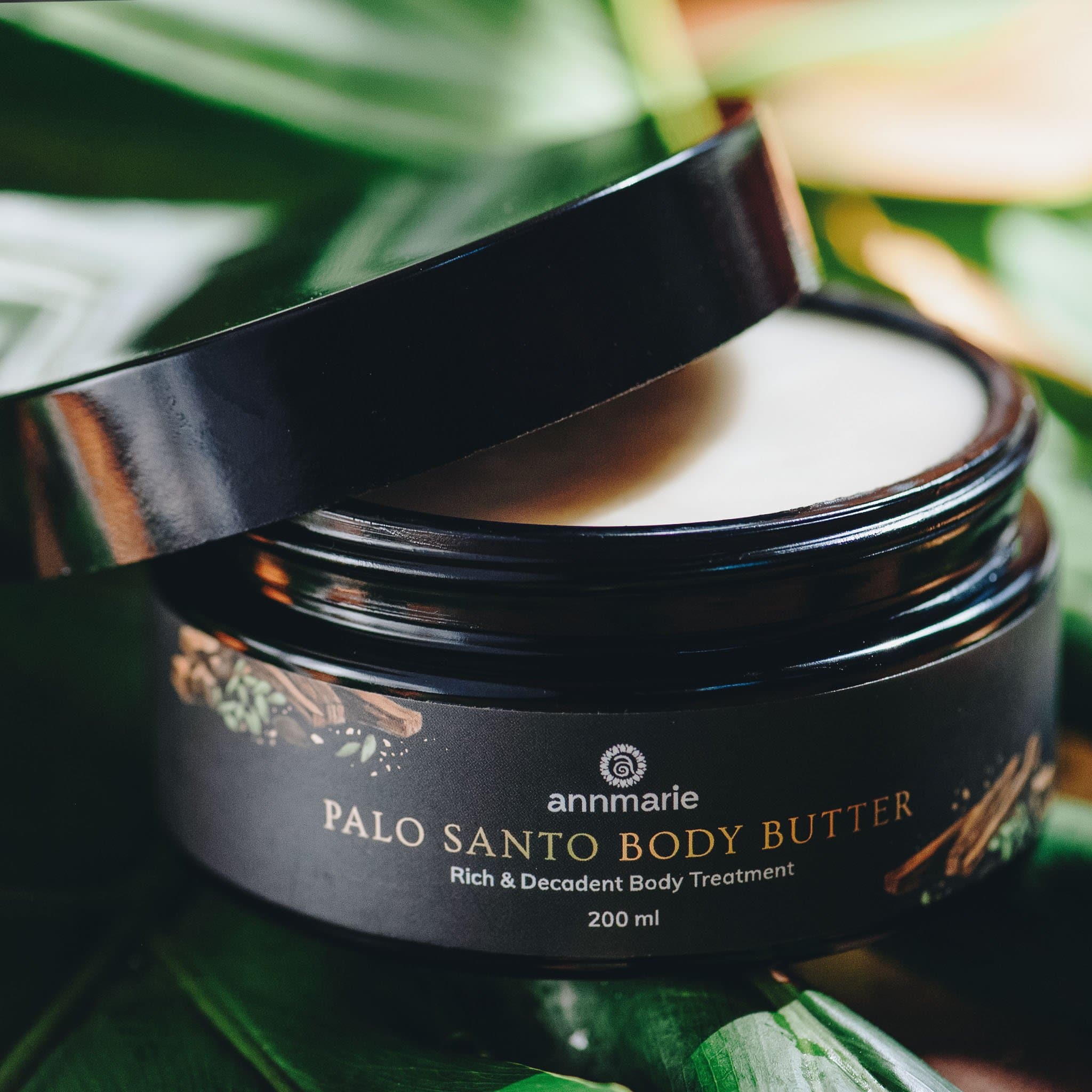This image is a meticulously staged product photo likely designed for a magazine or a small business website. It features a luxurious black jar of Palo Santo Body Butter, a rich and decadent body treatment, containing 200 milliliters of product. The jar is displayed against a backdrop of lush green foliage, possibly banana or palm leaves, giving the scene a tropical and spa-like ambiance. The jar itself is wide and short, with a black label that reads "Anne Marie" at the top, indicating the brand. The label's text is mostly white, with "Palo Santo Body Butter" in a goldish-yellow font. The lid of the jar is slightly tilted, leaning against the jar's left side, revealing the white, solid-like body butter brimming at the top. Additional decorative elements on the label, perhaps images of the natural ingredients used in the body butter, add to the product's artisanal and luxurious appeal.